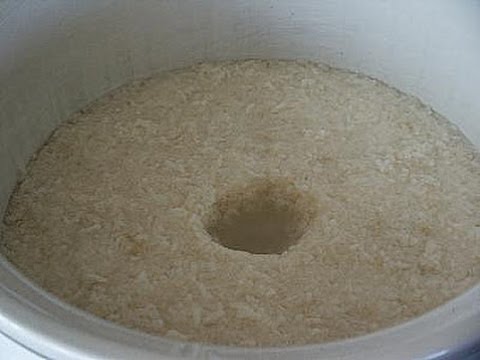The image depicts a close-up view of the inside of a container that is likely made of ceramic or glass, with the primary focus on its contents. Dominating the center of the image is what appears to be uncooked white rice, possibly soaked in water, giving it a slightly translucent appearance. There's a noticeable divot or hole in the center of the rice mound, which might be slightly off-center. There's very little color variation in the image, primarily featuring shades of white, off-white, tan, and a small amount of clear. Some hints of blue can also be spotted in the lower right-hand corner. The container has a distinguishable lip, suggesting that it might be a bowl or bucket. The setting and context are ambiguous, potentially indicating a restaurant environment or a basic storage setup possibly in a less affluent area. The image is somewhat grainy, complicating the exact identification of the materials and the setting.